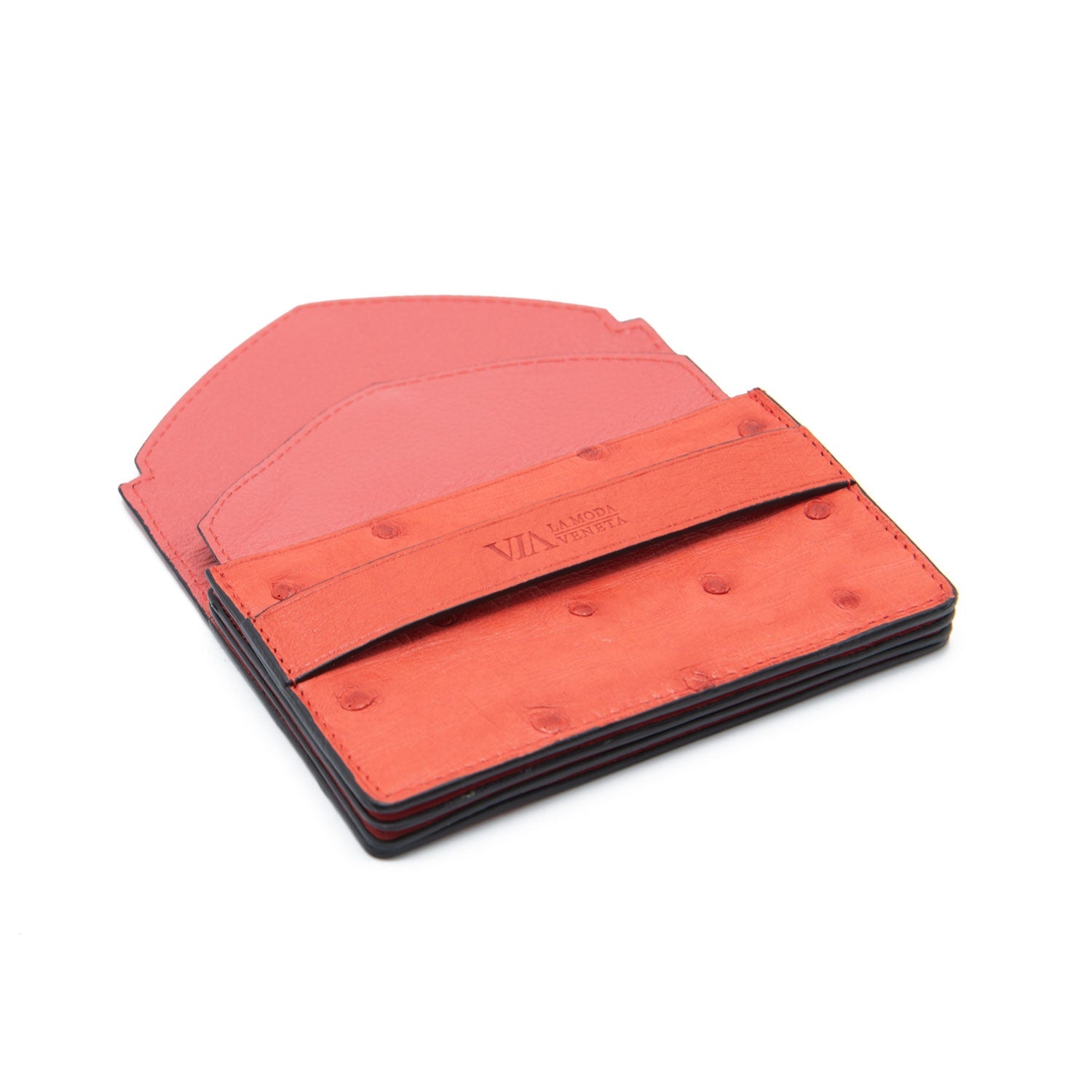The vertical image depicts a detailed and ornate accessory, likely a vintage-inspired purse or wallet, crafted from leather that exhibits a vibrant orangey-brown hue, transitioning into a slightly pinker shade within the interior. The design features accordion folds, allowing it to expand and accommodate more items. The exterior is adorned with small, decorative round indentations or metallic studs, adding to its intricate appearance. A prominent leather strap secures the front flap, embossed with a partially visible inscription that seems to include the characters “V/A” or possibly “VIA," which may reference "La Moda Veneta" or Venetian fashion. The flap is opened in the image, revealing an empty interior, indicative of multiple leather compartments and pockets designed for storage. The photograph is set against a simple white background, enhancing the purse's distinct colors and textures.